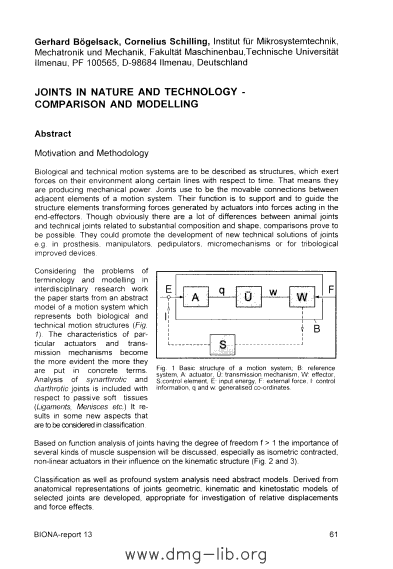This vertical rectangular image appears to be an excerpt from a scientific manual or textbook, featuring a white background and black print. The primary heading in bold text reads, "Joints in Nature and Technology: Comparison and Modeling." Just below, smaller bold text reads, "Abstract," followed by a section titled "Motivation and Methodology." The article underneath is authored by Gerhard Vogelsack and Cornelius Schilling from the German institution, Institut für Mikrosystemtechnik, Mechatronik und Mechanik, Fakultät Maschinenbau Technische Universität Ilmenau. The page includes detailed paragraphs and a complex diagram on the right side, labeled with various letters such as E-A-Q-O-W-W-S-B, possibly representing an algorithm. The diagram illustrates the basic structure of a motion system, including components like a reference system, actuator, transmission mechanism, effector, control element, input energy, external force, control information, and generalized coordinates. At the bottom of the page, the website www.dmg-lib.org is displayed, indicating the source of the document.